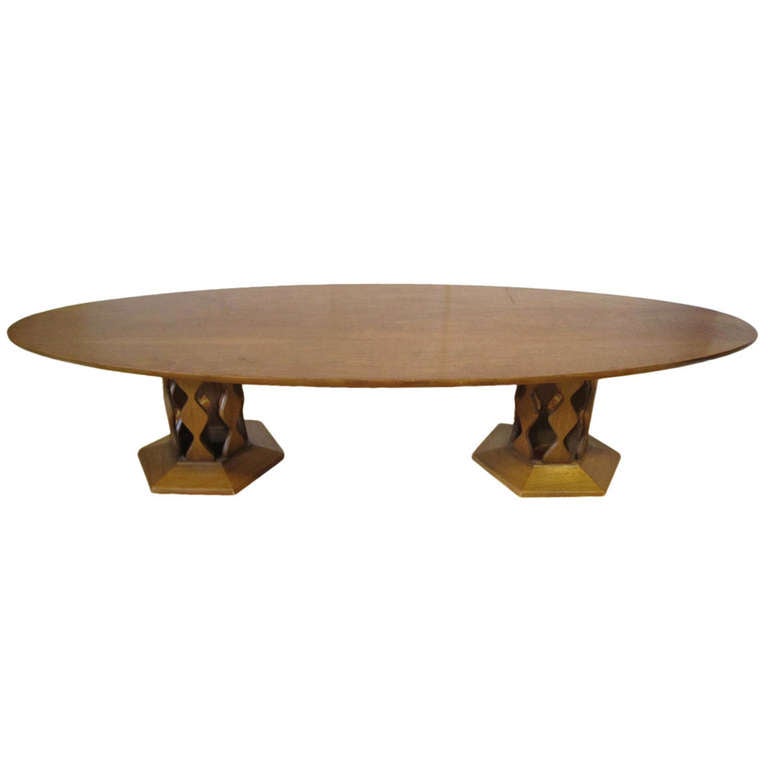This image showcases a uniquely designed coffee table that would fit right into the catalog of the Home Shopping Network or similar household item magazines. The table features a light brown, oval-shaped wooden top that resembles a surfboard or skateboard, lending a touch of modern quirkiness to its design. The table is supported by two short, stubby legs, each crafted from wood with a combination of dark brown and gold tones, although they might seem mismatched to some eyes. These legs are adorned with triangle patterns and have hexagonal bases that add a geometric flair. Despite its aesthetic appeal, the table appears to lean slightly to one side, indicating that one of the legs may not reach the ground fully, which could be a point of consideration for potential buyers. This low-to-the-ground coffee table would serve well as a stylish display piece for a cake, statue, or other decorative items. Additionally, these legs can seemingly be unscrewed if desired. The table is displayed against a neutral white backdrop, further emphasizing its distinct design features.